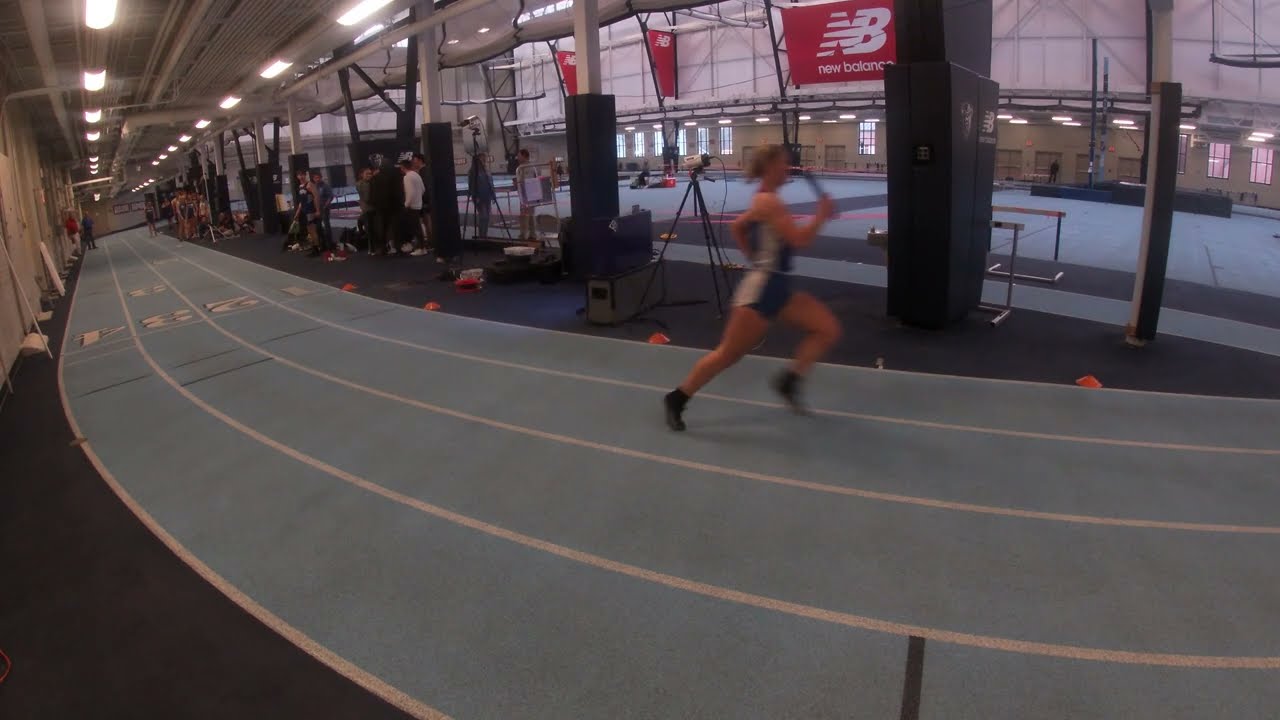In this detailed indoor scene, we are inside a large sports recreational complex featuring an indoor track field. The light blue track, distinctly marked with white lines dividing four lanes numbered 1 through 4, is the focal point. A woman in a track uniform is jogging around the track, gripping a baton in her hand. Surrounding her, multiple people are positioned, adding to the lively atmosphere. Prominent red New Balance flags and signs are displayed in the background, contributing vibrant color to the photo. The facility is well-lit by numerous white fluorescent lights, and blue and dark black pillars support the structure. An adjacent field of blue artificial turf serves as a recreation area. Multiple windows line the building, suggesting the photo was taken during the day. The vivid details highlight this indoor sports arena's functionality and energetic ambiance.